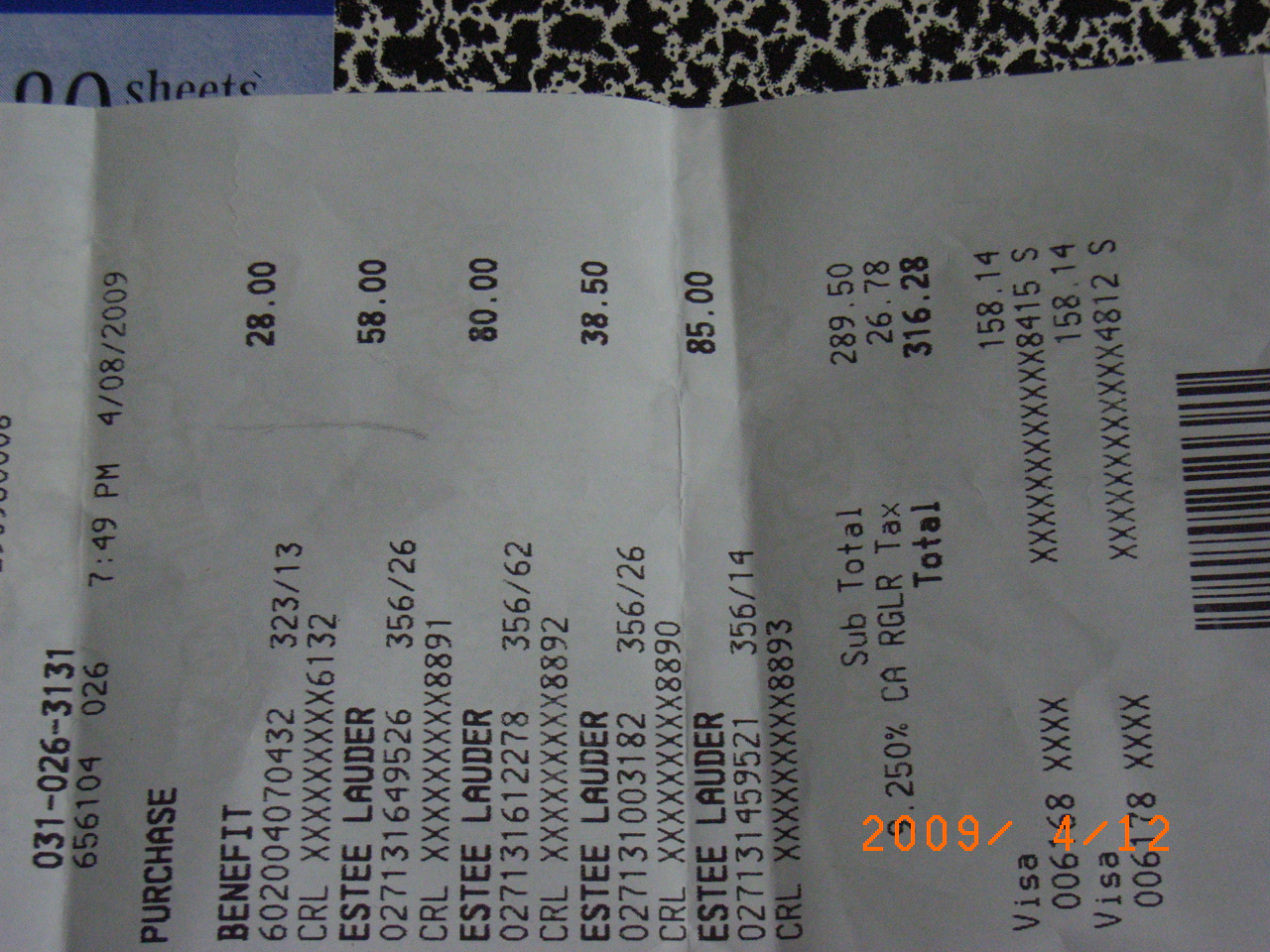The image captures a black and white receipt photographed on April 12th, 2009, with this date displayed in orange on the bottom right corner, typical of digital camera timestamps. The receipt is horizontally laid across what appears to be a black and white composition book, revealing part of its patterned cover. The receipt includes details such as a barcode at the bottom, and text in black lettering with various numbers: "031-026-3131" and "656104026". It lists a purchase time of 7:49 p.m. and a transaction date of April 8, 2009. The items listed on the receipt include one benefit product priced at $28, and four Estee Lauder products priced at $58, $80, $38.50, and $85 respectively. The subtotal is recorded as $289.50 with taxes amounting to $26.78, bringing the total to $316.28. The transaction was split across two Visa payments.